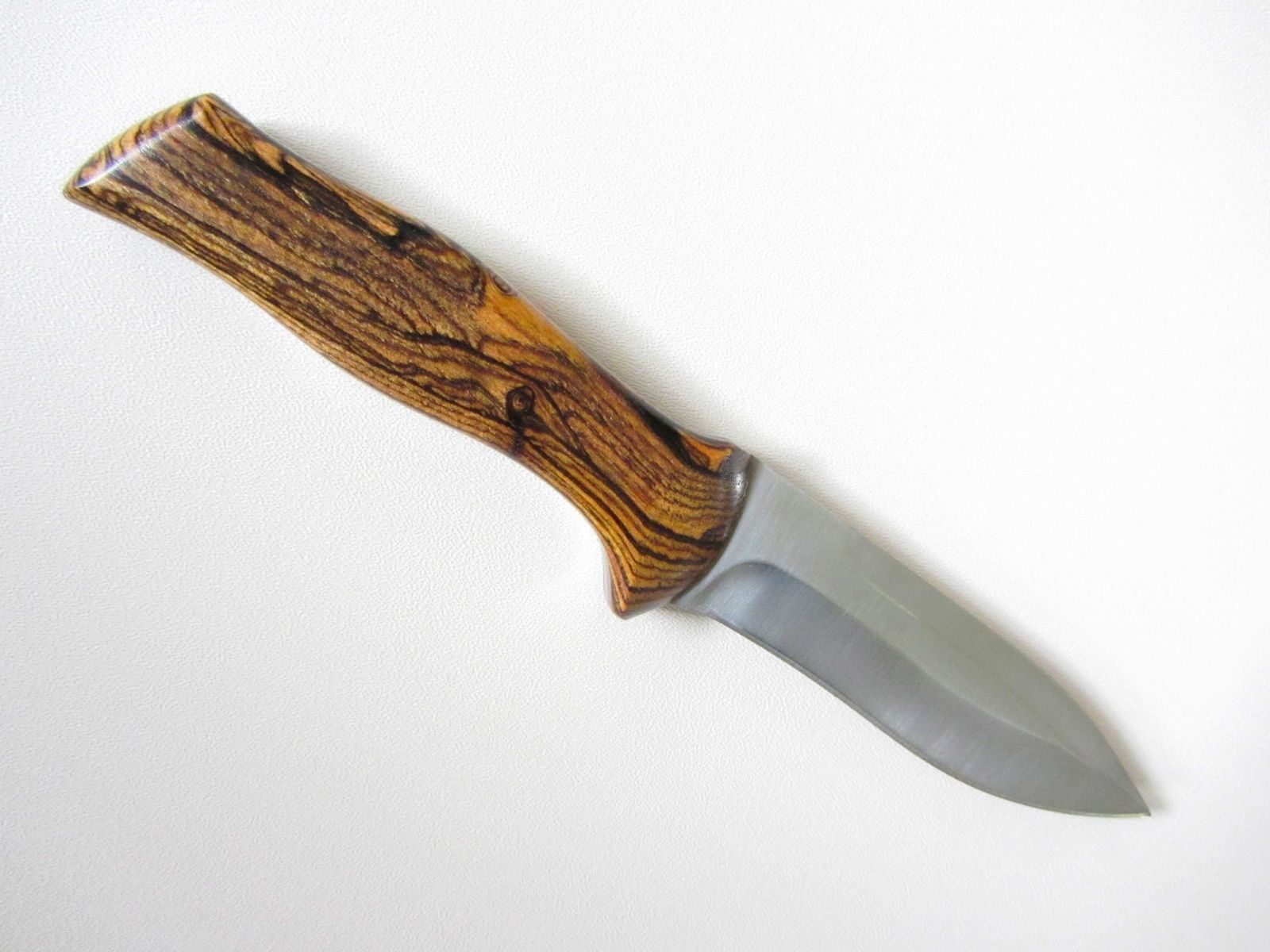This image displays a small hunter's knife set against a spotless white background, viewed from a top-down perspective. The knife is diagonally oriented, with the blade pointing toward the bottom right corner and the hilt angled toward the top left. The blade, crafted from stainless steel, is notably short, sharp, and curves slightly along the bottom edge, tapering to a fine point. The handle, featuring a finger stop for added safety, is made of light-colored wood accented with darker green and black grain patterns. The polished wood handle, which is contoured to fit comfortably in the hand, has a lacquered or waxed finish that gives it a subtle shine.